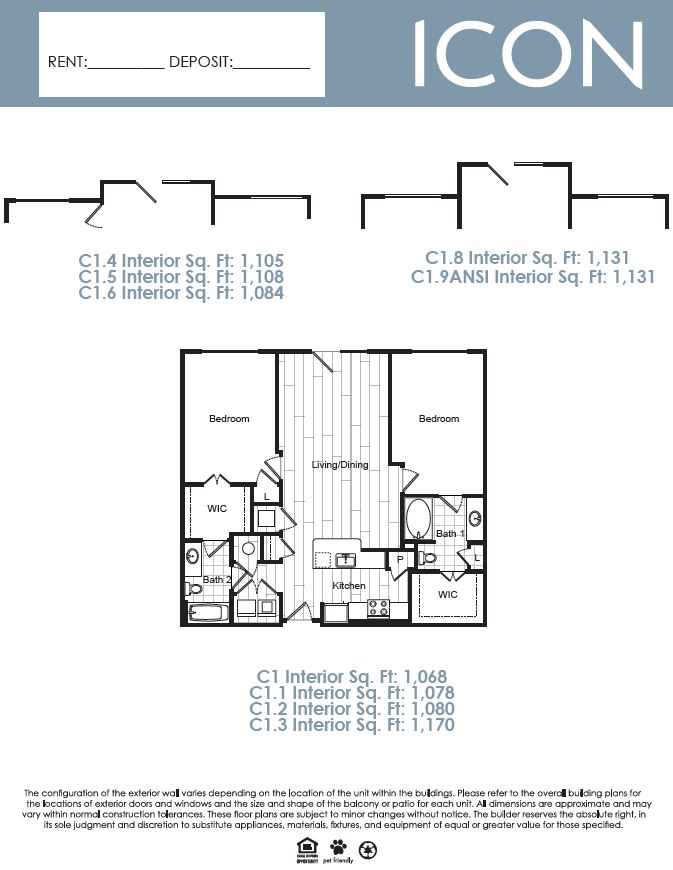**Detailed Description of a Two-Bedroom Apartment for Icon**

This image provides an illustrative floor plan and detailed rent information for a two-bedroom apartment offered by Icon. At the top of the image, the company's logo and rental details are prominently displayed. The logo “ICON” is written in bold, white, all-caps letters inside a blue-gray rectangular box. Adjacent to this, on a white rectangular background, the terms "Rent" and "Deposit" are shown in black text, positioned side by side.

The central part of the image features detailed door diagrams, accompanied by specific interior square footage dimensions for various layouts:

- **C1-4 Layout**: 1,105 sq. ft.
- **C1.6 Layout**: 1,108 sq. ft.
- **C1.8 Layout**: 1,131 sq. ft.
- **C1.9 ANSI Layout**: 1,131 sq. ft.

These measurements are displayed vertically above each respective door diagram.

To the right, the image showcases a comprehensive floor plan of the two-bedroom apartment. The bedrooms are located on the upper left and upper right corners of the layout. Each bedroom includes distinctive features:
- The bedroom on the upper left features a walk-in closet and is connected to a bathroom (Bath 1).
- The bedroom on the upper right boasts a master bathroom and a much larger walk-in closet.

Between the two bedrooms lies the shared living and dining area. This central space includes an island-style counter that extends outward from the right wall, housing a sink. The stove and refrigerator are strategically placed against the back wall.

Additional features of the floor plan include:
- **Bath 1** and **Bath 2**: Standard bathrooms placed near each bedroom for convenience.
- **Washer and Dryer**: Located in a closet for easy laundry access.

The provided layouts and their corresponding interior square footages are indicated below each diagram in blue-gray text, ensuring that prospective renters have all necessary information at a glance.

Overall, the image is a comprehensive guide for individuals interested in renting a two-bedroom apartment from Icon, offering clarity on the apartment's layout, amenities, and space utilization.